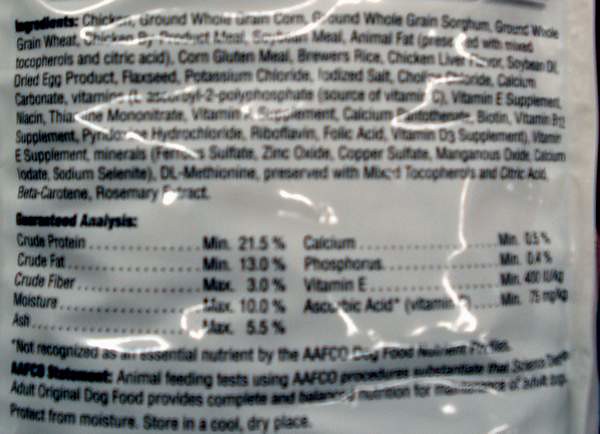The back of a food product package is captured in a highly reflective white plastic material, causing some text to blur due to glare. Despite this, the ingredients list is partially legible. It includes chicken, whole grain corn, ground whole grain sorghum, ground whole grain wheat, chicken by-product meal, soybean meal, animal fat, corn gluten meal, brewers rice, chicken liver flavor, soybean oil, dried egg product, flax seed, potassium chloride, iodized salt, biotin, vitamin B12 supplement, hydrochloride, riboflavin, folic acid, vitamin E supplement, minerals, DL-methionine, mixed tocopherols (preservative), citric acid, beta carotene, and rosemary extract. Nutritional information on the package specifies crude protein at 21%, crude fat at 13%, crude fiber at 3%, moisture at 10%, ash at 5.5%, calcium at 0.5%, phosphorus at 0.4%, vitamin E at 400 IU/kg, and ascorbic acid (vitamin C) with a minimum of 75 mg.